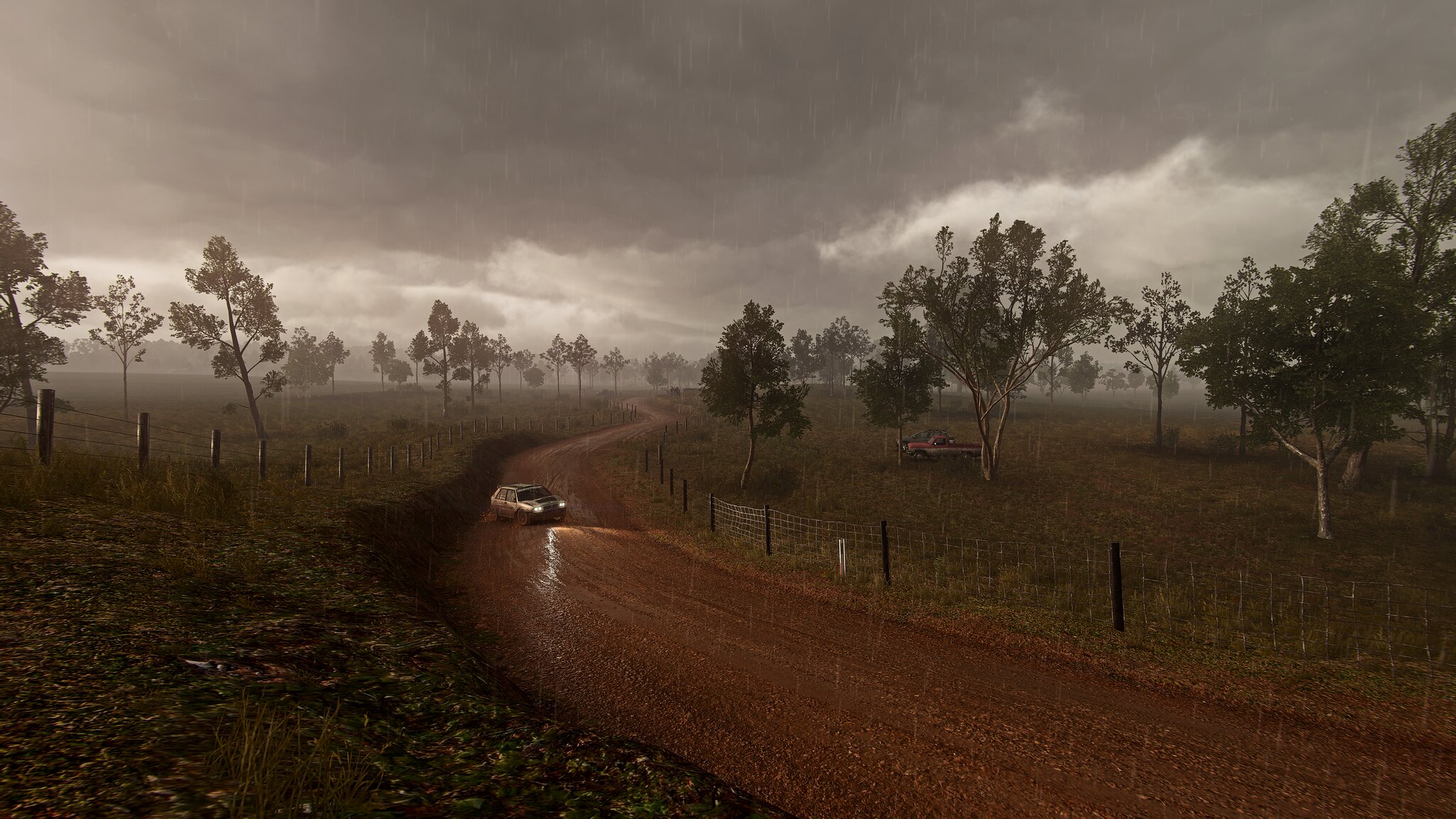A car navigates a wet, muddy dirt road, its headlights casting a reflective sheen on the slick surface. Positioned midway down the road, the vehicle appears slightly askew, suggesting it may have either skidded or is preparing to turn around. Flanking the road are wire fences that delineate the boundaries of surrounding fields. Dense clusters of trees with prominent trunks occupy these fields, and an old pickup truck, seemingly abandoned with no clear path leading to it, sits idly in the field to the right. The sky overhead is dark and heavily clouded, intensifying the dreary atmosphere. Weeds proliferate along the roadside, adding to the sense of neglect and ruggedness.